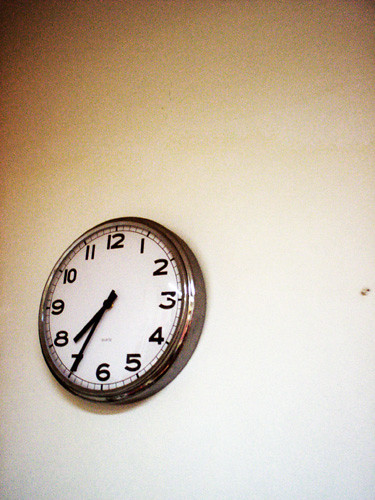This image is a portrait-oriented photograph of a simple, traditional-looking clock mounted on a predominantly white wall. The wall exhibits varying shades due to the lighting, and the clock is positioned off-center, towards the lower-left portion of the image. The clock features a white face with black, traditional-style numerals and black hands, with the hour hand being slightly thicker than the minute hand. It is encased in a brown frame, which could be either wood or metal. The time displayed is exactly 7:35. The photo appears to be taken from an odd angle, giving it a slightly skewed and off-center perspective, emphasizing the utilitarian and minimalist nature of the clock against the stark white background. There's nothing else in the picture to distract from the focus on the clock.